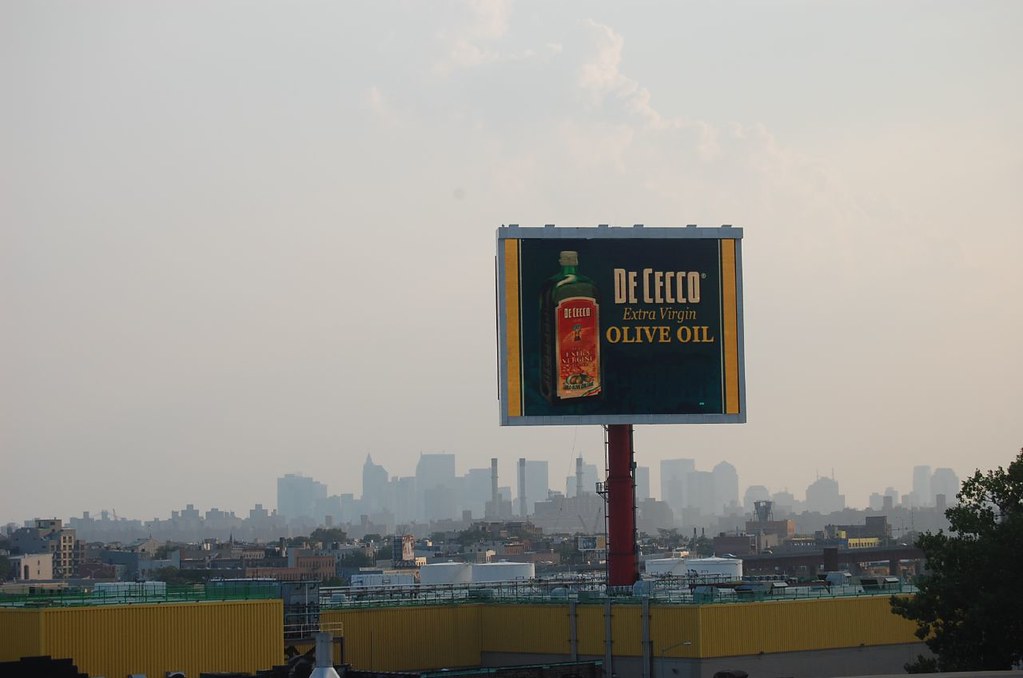Aerial view photograph of a bustling cityscape, likely captured from a high vantage point such as a rooftop or a high window. The perspective offers a striking view straight across the tops of several tall buildings. In the background, the skyline recedes into a gray, misty atmosphere, with the tall structures partially obscured by fog, creating an ethereal and moody ambiance. The midground is populated with numerous factory-like buildings, adding an industrial touch to the scene. 

In the forefront, a prominent yellow building stands out with its rooftop rim accentuating its position. The building itself is predominantly gray. Towards the top middle-right of this structure, a striking red pole with scaffolding attached to it captures the eye. Adjacent to the red pole is a large rectangular sign with a gray metal trim. The sign's left and right edges are highlighted in yellow, and it features a dark background. 

On the left side of the sign, a jar with a white lid and a red label can be seen, prominently displayed. To the right on the sign, in bold white letters, it reads "D.E.C.E.C.C.O." Below this text, in yellow letters, it states "Extra Virgin," followed by "Olive Oil." This detailed signage adds a commercial element to the urban landscape, blending modern corporate aesthetics with the surrounding architecture.